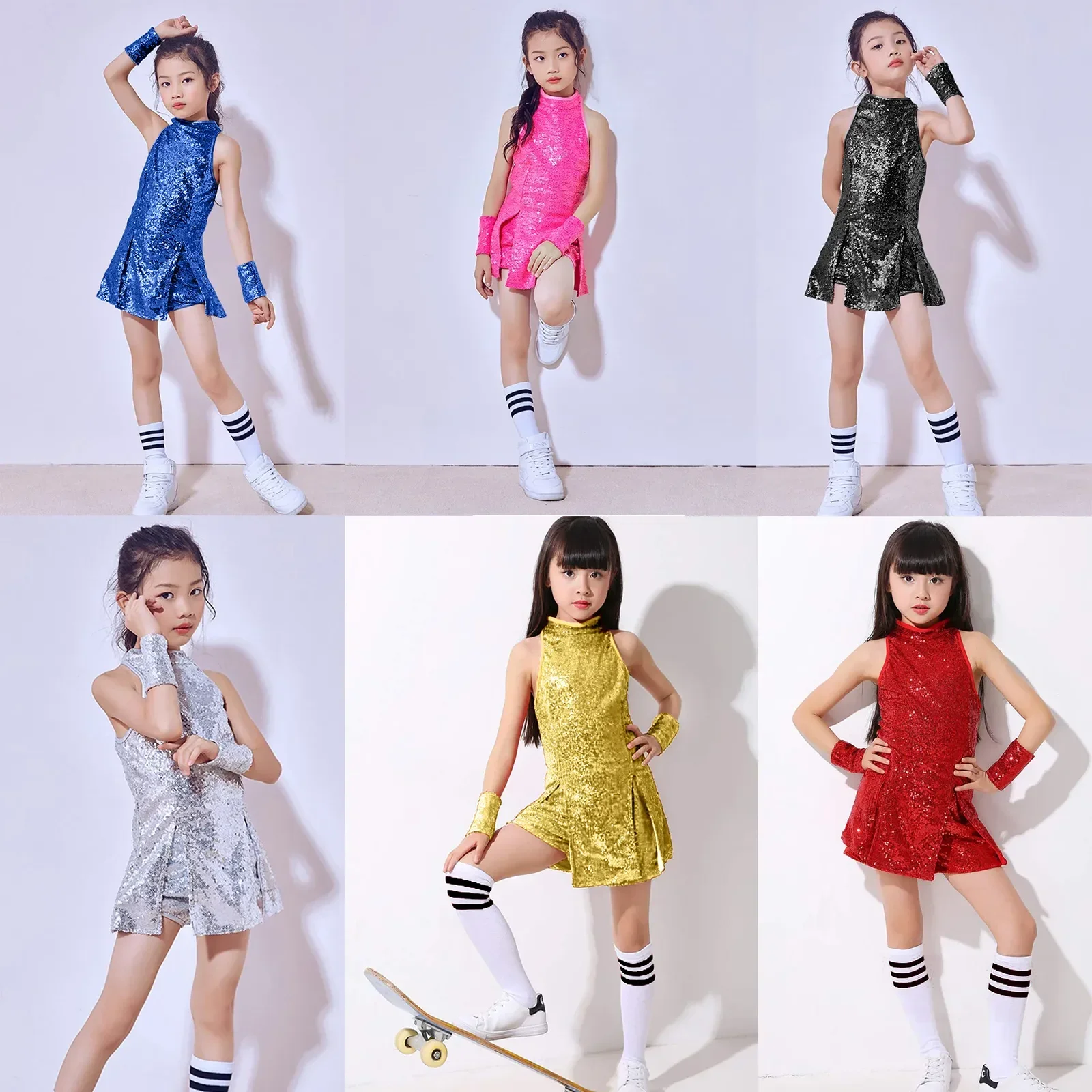The image is a composite of six photographs featuring a young Asian girl modeling in various outfits. Each outfit is a different color of a similar dress style, resembling cheerleader dresses. She is consistently wearing white socks with black stripes and white shoes. Her black hair is styled differently in some of the images. In the top row, she is wearing a sparkly blue dress with matching wristbands in the top left, a pink dress in the top middle, and a dark greenish-black dress in the top right. In the bottom row, she appears in a silver dress on the bottom left, a yellow dress in the bottom middle, and a red dress in the bottom right. The backdrop is a simple wall and floor, suggesting an indoor setting. Notably, she's facing forward in all images, and one photograph even shows her on a skateboard. Each dress is accessorized with wristbands that match the color of the dress, adding a subtle yet cohesive detail to her overall look.